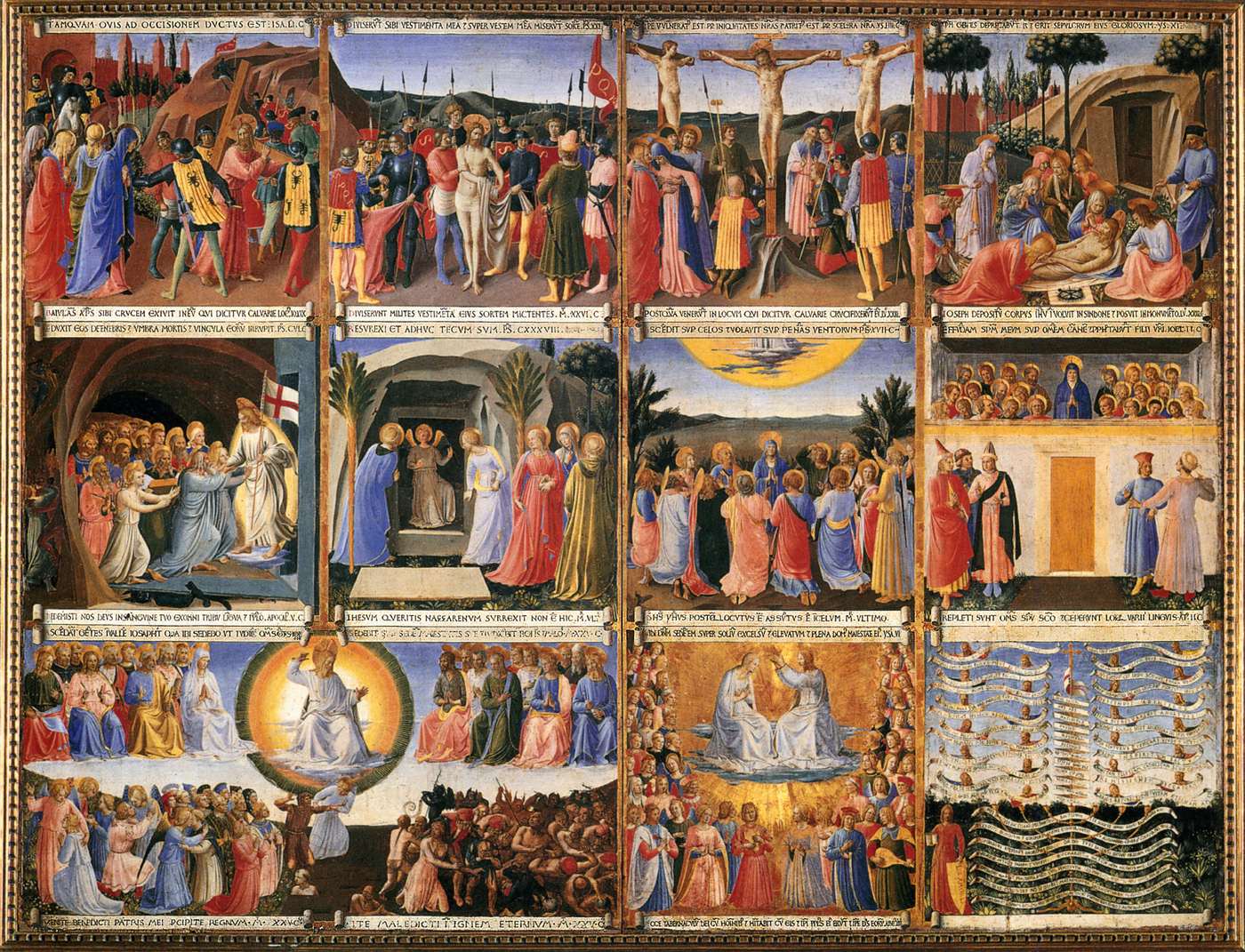A vibrant and richly detailed medieval-style artwork, presented as a collage of 12 square scenes laid out in a 4x3 grid, each capturing a dramatic moment from the biblical narrative of Jesus Christ. Each image is meticulously labeled in an ancient language, perhaps Roman or Latin. The top row begins with Jesus, fully clothed, being carried by men adorned in capes with scorpion emblems. This is followed by scenes of Jesus disrobing, the crucifixion featuring three crosses, and finally his body being laid out on the ground. The second row starts with Jesus surrounded by a crowd, standing before a white flag with a red cross, an image of a cave with an angel and people outside, a group kneeling in prayer, and a depiction of a courtroom-like setting. The last row includes interconnected scenes showing people gazing upwards towards a central image of Jesus encircled in the sky, Jesus crowning a woman while surrounded by celestial beings, and concludes with banners displaying names of various figures. The imagery, steeped in historical and religious symbolism, suggests a narrative arc from Jesus' crucifixion and entombment to his resurrection and ascension.